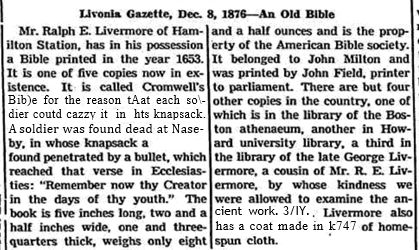The image depicts an article from the "Livonia Gazette" dated December 8, 1876, titled "An Old Bible." The article, printed on a white background with black borders dividing it into two columns, details a historical account centering on a rare Bible. The first column informs that Mr. Ralph E. Livermore of Hamilton Station possesses a Bible printed in 1653, known as Cromwell's Bible because soldiers carried it in their knapsacks. Notably, one such Bible was found with a deceased soldier at the Battle of Naseby, the bullet having stopped at the verse in Ecclesiastes: "Remember now thy creator in the days of thy youth." The book's dimensions are five inches long, two and a half inches wide, and one and three-quarters inches thick, weighing eight and a half ounces. The second column continues, noting that the Bible is owned by the American Bible Society and once belonged to John Milton. It was printed by John Field, Printer to Parliament. Only four other copies exist, located in the Boston Athenaeum, Harvard University Library, and the library of the late George Livermore, Mr. Ralph E. Livermore's cousin. Additionally, Ralph E. Livermore owns a coat made of homespun cloth marked "K747," underscoring the article's emphasis on the preservation of significant historical artifacts.